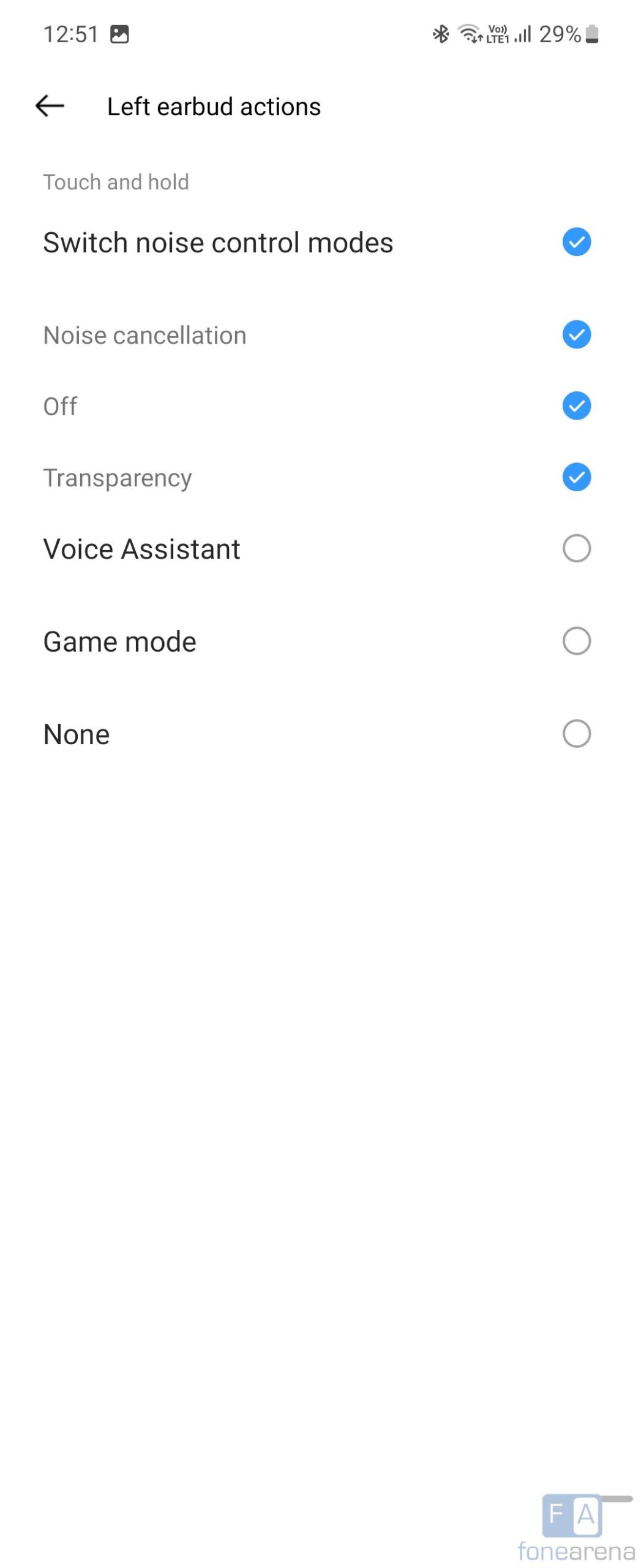This image is a detailed screenshot from PhoneArena, displayed in portrait mode. At the bottom right corner of the screenshot, the logo for PhoneArena is visible, featuring an "F" on a blue background and an "A" on a white background, resembling a toggle switch. 

At the top left corner, the time is shown as 12:51. In the upper right, the battery icon indicates a 29% charge, suggesting the screenshot was taken on a cell phone.

Below the top bar, the interface shows various settings for configuring a left earbud's functionality. The settings begin with a row displaying a back arrow and the label "Left Earbud Actions". 

The subsequent rows feature the following details:
- The text "Touch and Hold" displayed in gray on white, with difficulty in readability.
- "Switch Noise Control Modes" with a blue checkmark indicating it is selected.
- "Noise Cancellation" with a blue checkmark indicating it is selected.
- "Off" with a blue checkmark indicating it is selected.
- "Transparency" with a blue checkmark indicating it is selected.
- "Voice Assistant" is listed with no checkmark.
- "Game Mode" is listed with no checkmark.
- "None" is listed with no checkmark. 

This screenshot from PhoneArena offers a comprehensive guide to selecting and configuring functionalities for your left earbud.